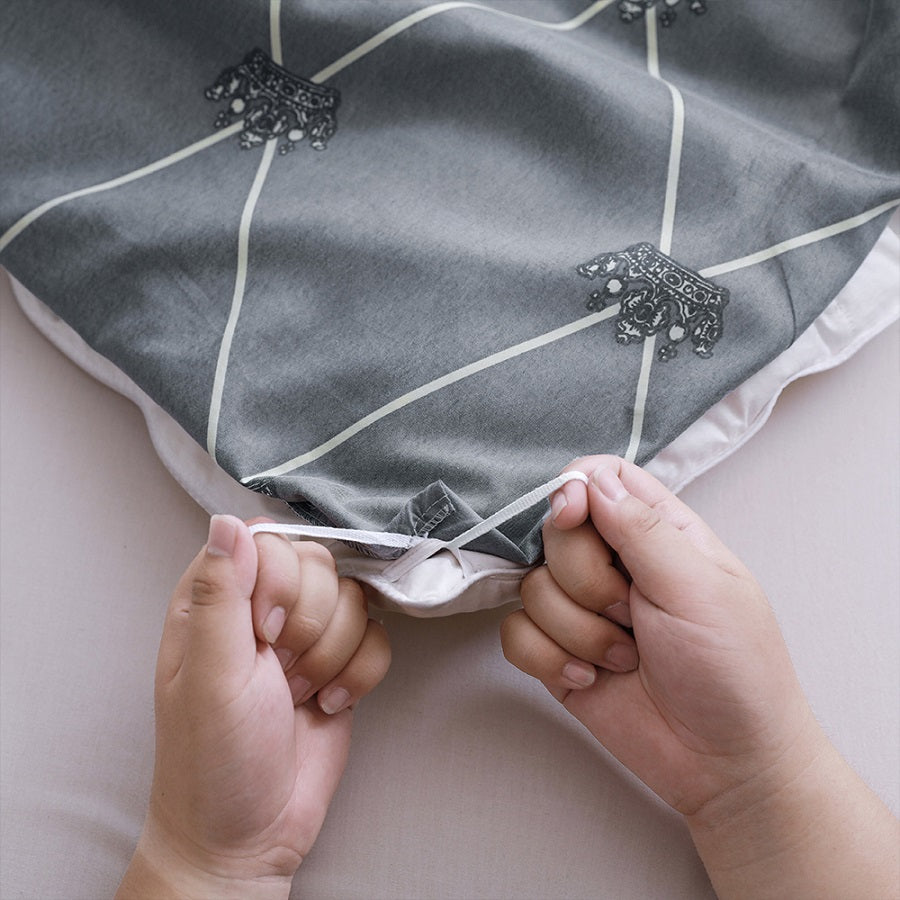In this detailed photograph taken indoors, we are looking down at a pair of hands, belonging to a person of Caucasian descent, as they tie a corner of a comforter. The hands, characterized by clean and slightly longer, polished nails, emerge from the bottom edge—one from the lower right corner and the other just to the right of the lower left corner. The fingers are slightly pudgy and curved as they skillfully handle the tying threads. 

The comforter itself, prominently positioned from the top of the image, is a light gray color adorned with white crisscrossing lines that meet to form X shapes. At each intersection, a white-filled crown bordered by black lines is depicted, adding an intricate design element to the fabric. This comforter extends about an inch from the top left and right sides down to form a visible corner toward the bottom center. The underside of the comforter is pink, resting against a matching light pink background, possibly a sheet or surface, creating a cohesive and soft visual palette.